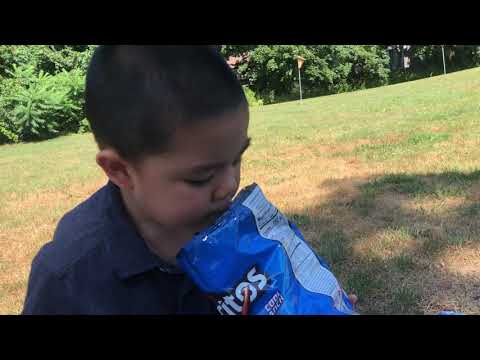In this outdoor photo, a young toddler-aged boy with a short haircut, round nose, and large ears, likely of Asian descent, is seated on sloping green grass with a brown patch in the foreground. He is holding an open bag of blue Doritos Cool Ranch chips, white nutritional information visible on the bag. Dressed in a buttoned-up blue shirt with a collar, the boy intently peers into the chip bag, his mouth and eyes focused. Behind him, the lush green foliage creates a vibrant backdrop. Shadows cast on the lawn suggest it is a bright, sunny day.